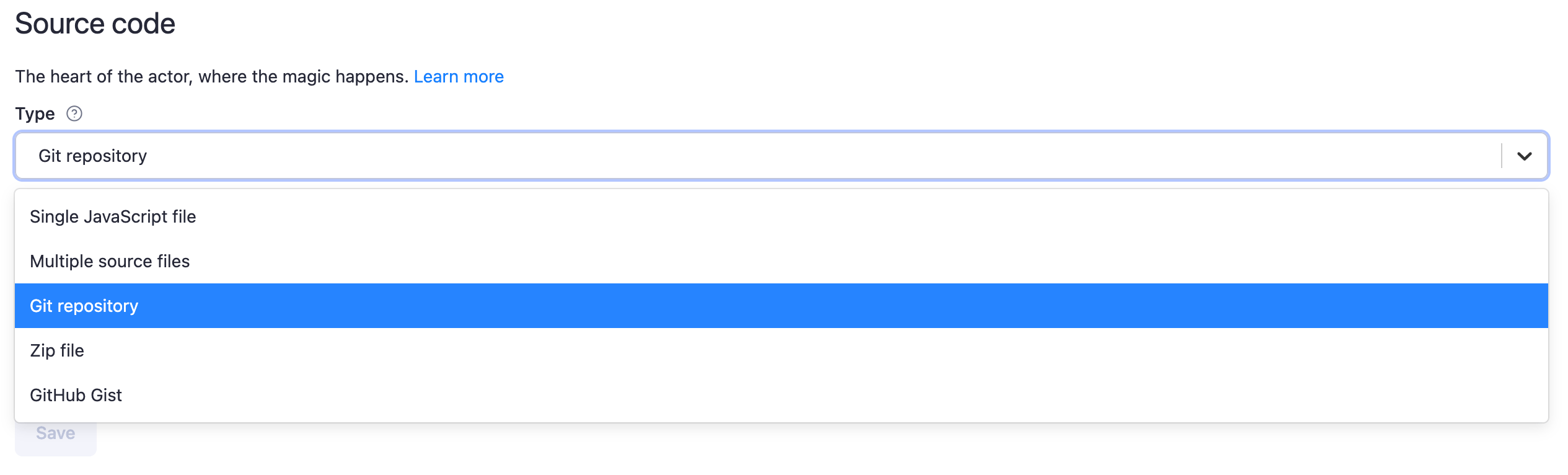This image is a screenshot of a website with a clean, white background. At the very top, in large black letters, the title "Source Code" is prominently displayed, with the "S" capitalized. Directly below the title, in smaller font, there is a subtitle that reads "The heart of the actor, where the magic happens." This is accompanied by a blue hyperlink labeled "Learn More."

Further down the page, the word "Type" is displayed with a question mark symbol next to it, indicating a prompt for user input. Underneath this prompt is a dropdown menu. The currently selected option in this menu is "Git Repository," which is highlighted in blue. The dropdown contains several other options listed from top to bottom: "Single JavaScript File," "Multiple Source Files," "Zip File," and "GitHub Gist." 

The dropdown menu is slightly overlaying the top part of a small "Save" button, which is colored a slightly dark grey. The "Git Repository" option being highlighted indicates that it is the active selection. The rest of the background remains a clean, unadorned white.